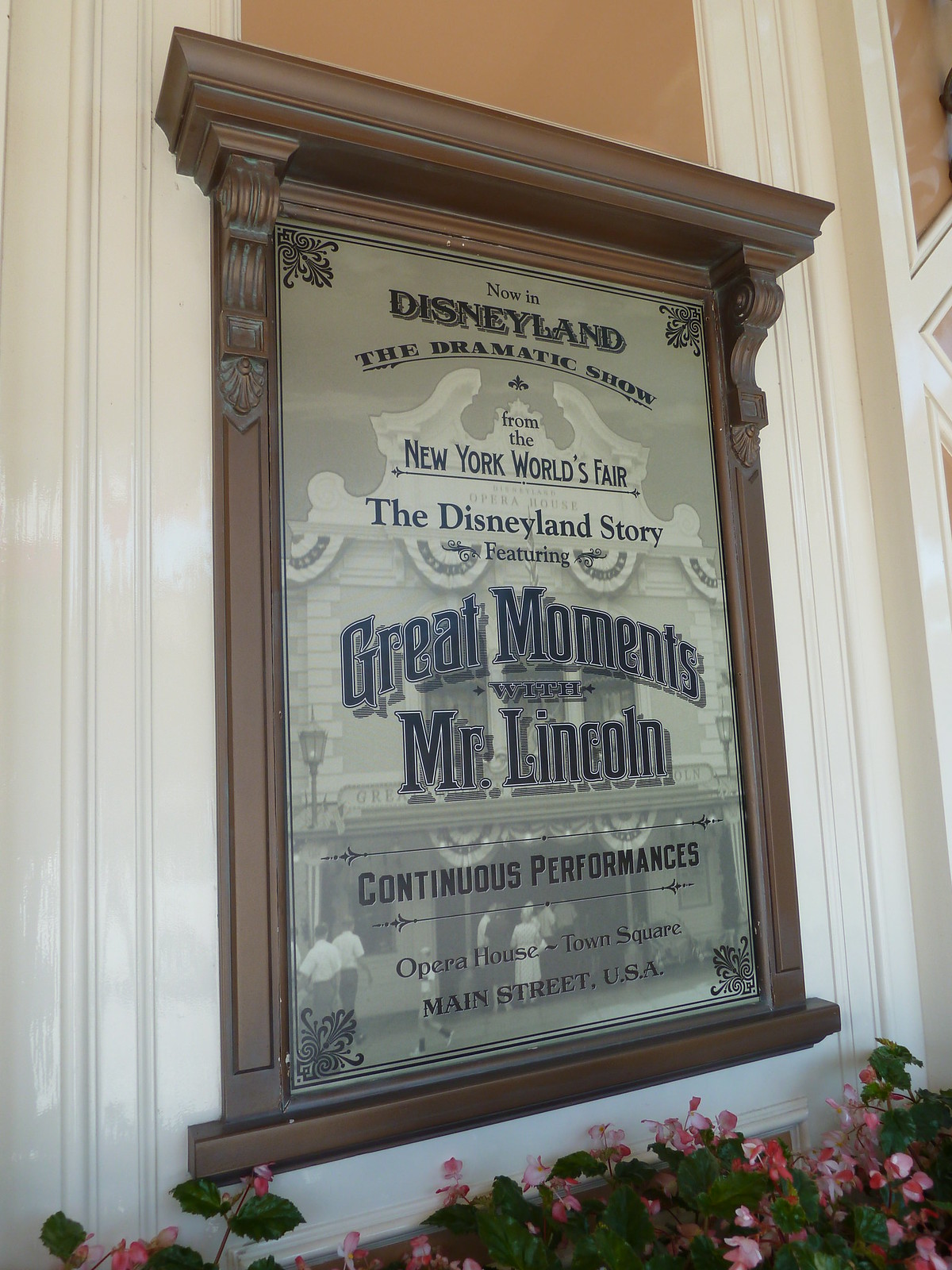The image depicts a framed sign outside an auditorium in Disneyland, advertising an ongoing event. The sign promotes "The Disneyland Story Featuring Great Moments with Mr. Lincoln," a dramatic show originally from New York's World's Fair, now presented with continuous performances at the Opera House in Town Square, Main Street, USA. The sign, encased in glass and bordered with intricately detailed brown wood, is about seven feet tall with bold black lettering on a white background. Below the sign is a flower bed of vibrant pink flowers, creating a welcoming entrance. The building itself has a white facade with some modern elements visible in the background.